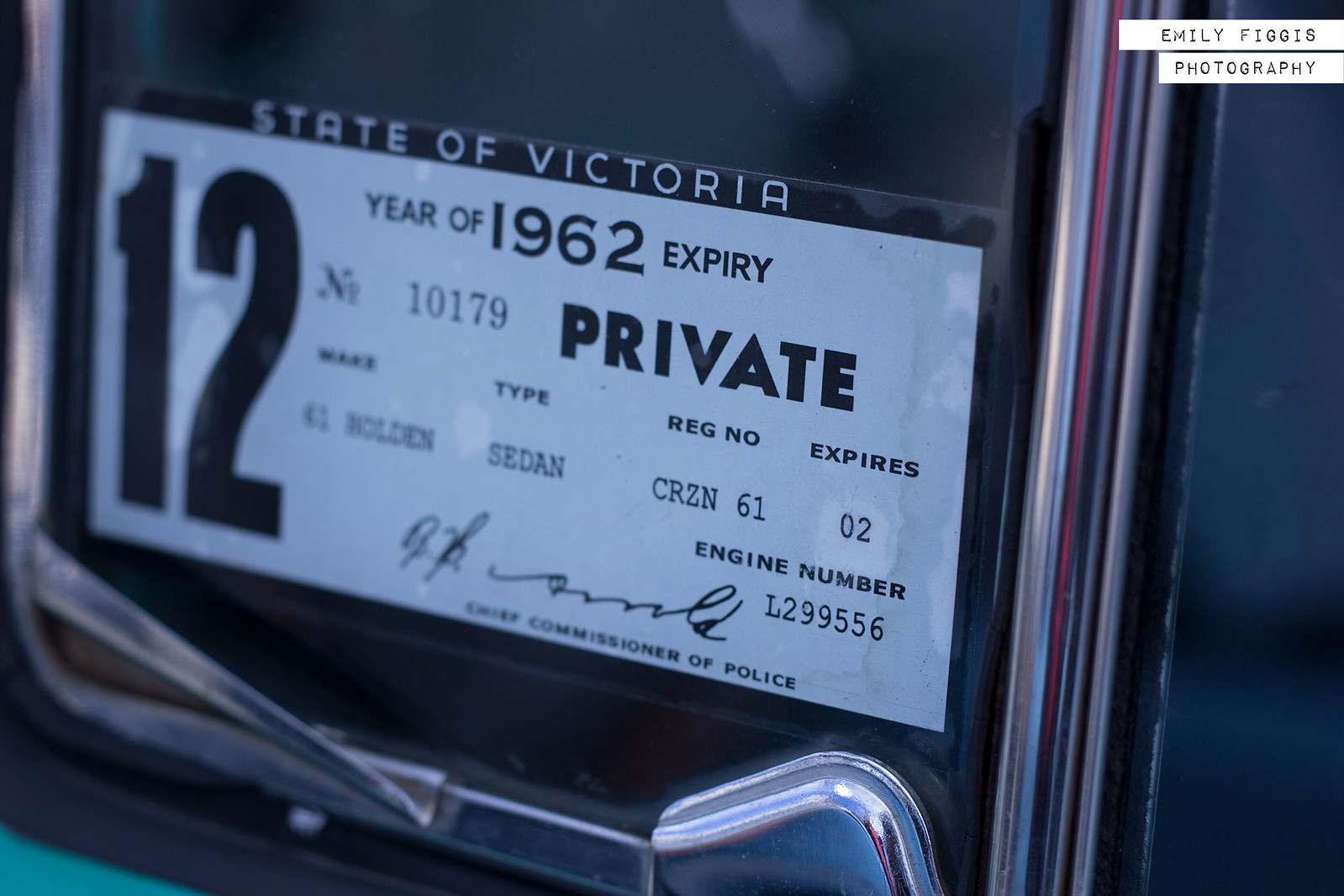This image depicts a close-up of a registration certificate affixed to a car's windshield. The windshield is bordered by a silver aluminum frame, with blue glass as the background. Centered at the bottom of the windshield is a horizontal rectangular sticker with a black border enclosing the text. The top of the black border prominently displays the words "State of Victoria" in white text. Inside the rectangle, the background is white, and on the left side, large numbers read "12." Adjacent to these numbers, several lines of black text provide details: "year of 1962," "Expiry number 10179," "Private," "make Holden," "type sedan," "registration number CRZN61," and "expires 02." Further down, the text includes "engine number L299556" and a signature, which is not legible, followed by the title "Chief Commissioner of Police." Additionally, the top right corner of the image features the watermark "Emily Figgis Photography." The registration sticker appears to be taped to the windshield with metal pieces visible underneath.